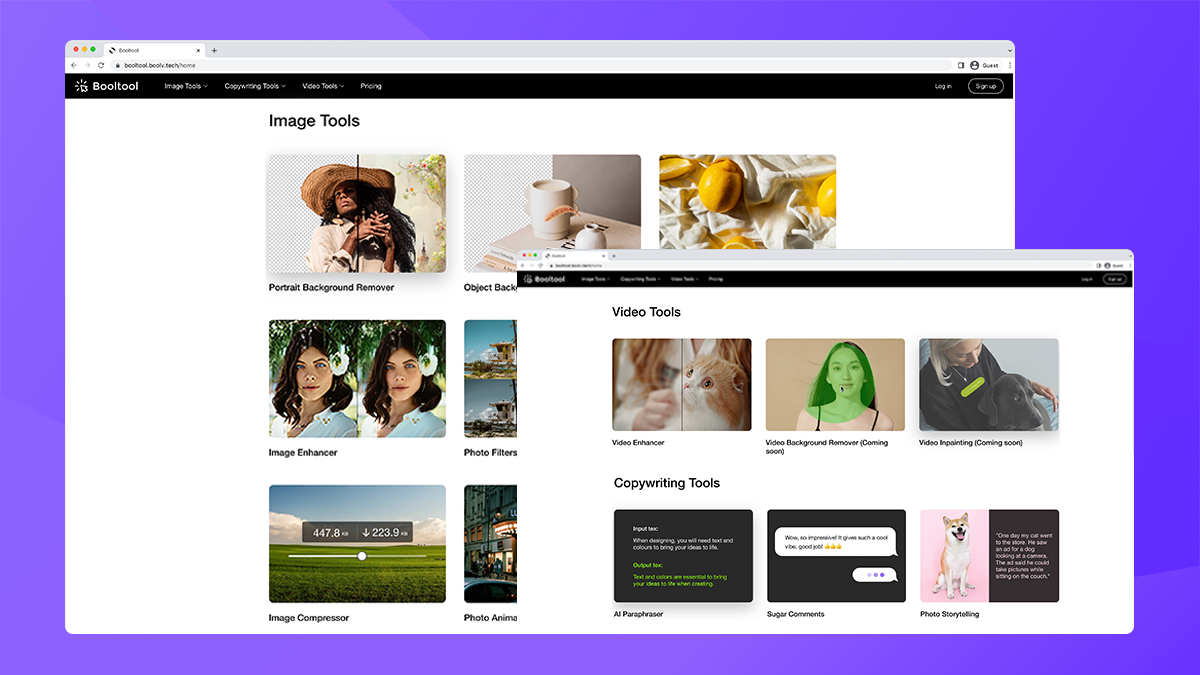The image features a layered display of two website pages against a collage of abstract purple shapes, which range from medium to dark purple hues. The two website pages share a similar design. Each page has a light gray header with red, yellow, and green circles arranged from left to right, followed by a light gray tab leading to another light gray header. This header contains left and right navigation arrows, a refresh button, and a long white URL bar with black text. Below this, a black header contains white text on the left that reads "Google Tool, BOOLTOOL," and on the right, there are four white text sections followed by "Log In". Additionally, there is a black button outlined in white with the text "Sign Up." 

The main content of the web pages diverges below the headers. While both pages feature rows of images each paired with bold black captions beneath, they serve different purposes. The larger page, occupying the left two-thirds of the frame, is labeled "Image Tools" in black text at the top left. Overlaid on top and partially extending over the purple background to the right is the smaller page, labeled "Video Tools" in black text at the top left. This composition highlights the primary focus on the "Image Tools" site while offering a glimpse of the related "Video Tools" page.